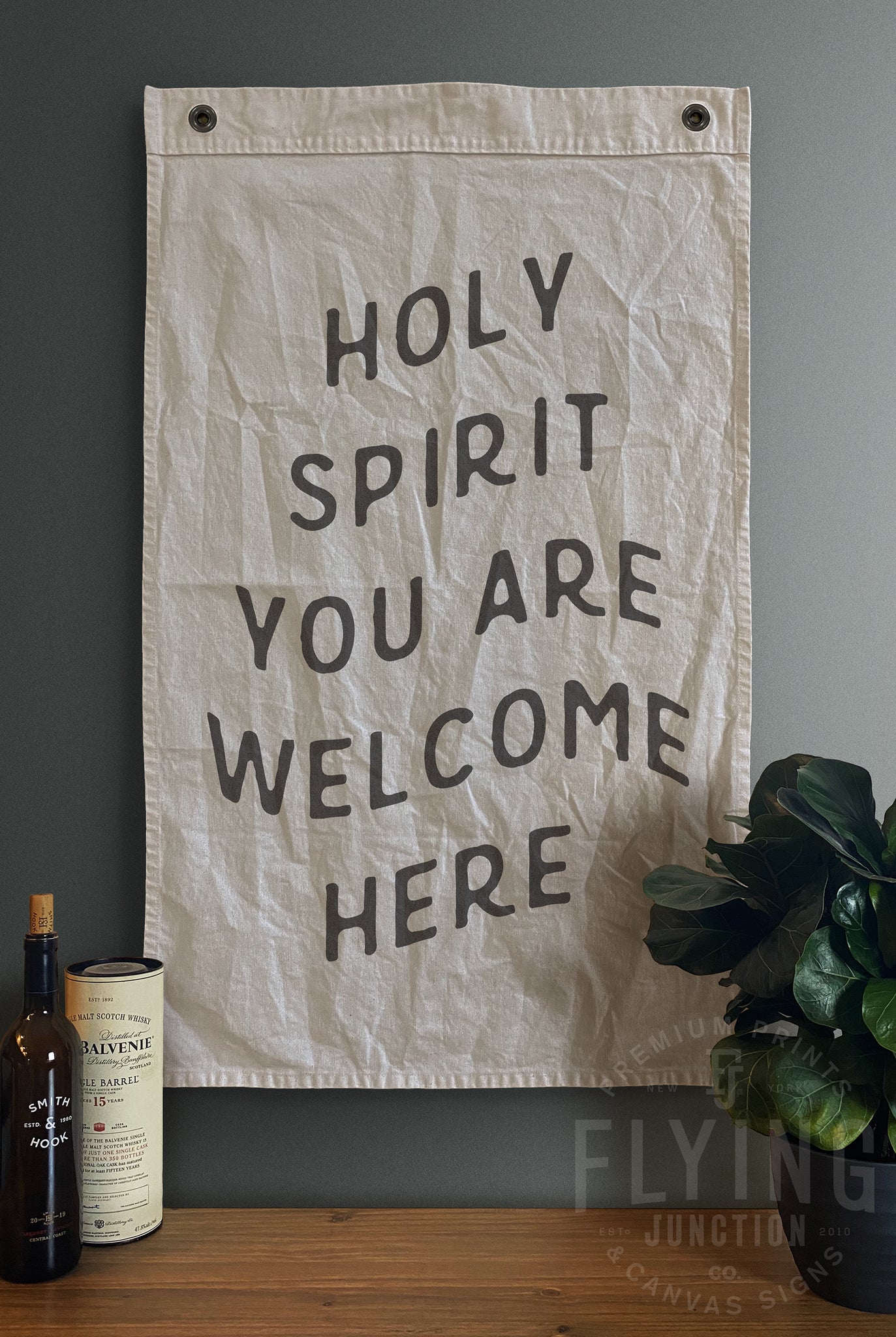The photograph, oriented in portrait mode, captures a detailed indoor scene. Dominating the image is a medium gray-painted wall, adorned with a white canvas poster that has two eyehooks for hanging. Centered on the poster, in prominent black text, are the words: "Holy Spirit, you are welcome here." Below the poster, a medium brown wooden table extends across the bottom of the image. On the left side of the table, there is a dark black bottle labeled "Smith & Hook" in white text, and another bottle labeled "Balvenie Scotch Whiskey." On the bottom right corner of the image, partially on the table, is a black pot containing a green plant, possibly a ficus. Additionally, a logo in light gray text reading "Premium Prints Flying Junction Co. and Canvas Signs" is faintly visible in the image’s lower right corner.